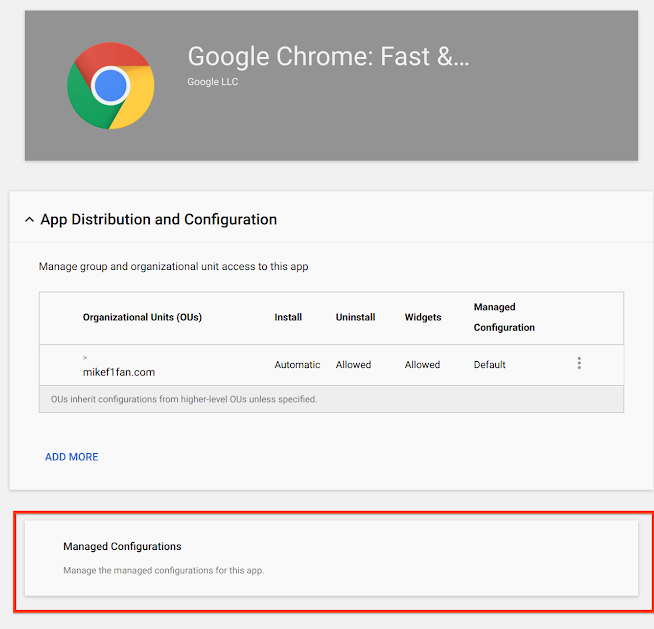This is a detailed description of a screenshot capturing the Google Chrome settings page. At the top, a gray banner stretches across the screen, prominently featuring the Google Chrome logo on the left side. The logo is circular, divided into three swirling sections colored red, green, and yellow, with a smaller blue circle at its center. To the right of the logo, the text reads "Google Chrome: Fast and..." in a clear font, followed by "Google LLC" in smaller white text beneath it. Below the banner, there is a lighter gray box containing a collapse button denoted by an up arrow. This section is labeled "Distribution and Configuration," and it specifies the management of group and organizational access to the app. Underneath this section, there is a table consisting of five columns. The columns are titled: Organizational Units (OUs), Install, Uninstall, Widgets, and Managed Configuration.